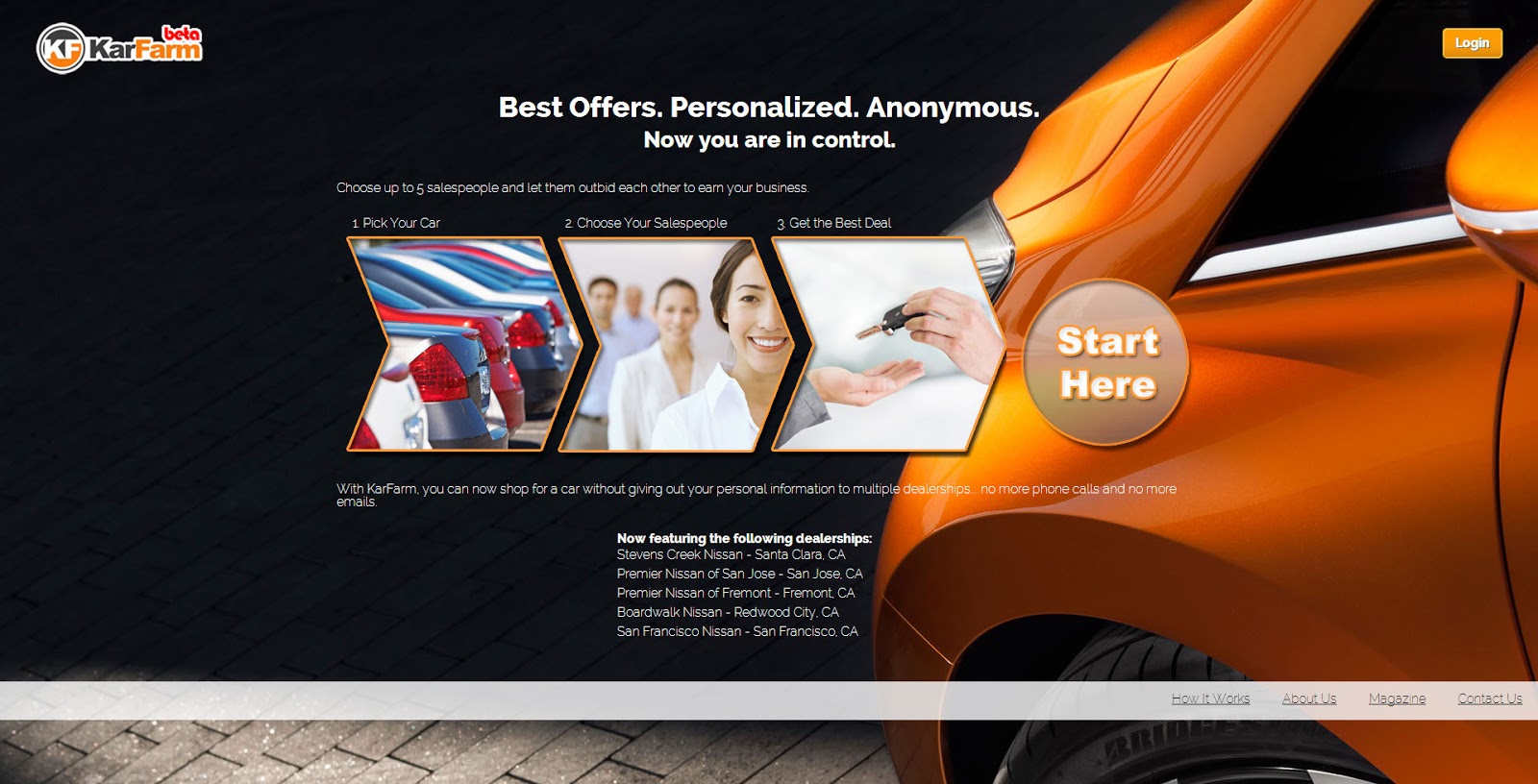**Image Description:**

The image features a sleek black background. In the top left corner, there is a circular logo with the initials "KF" and the text "Car Farm." To the top right, there is an orange button labeled "Login."

Centrally positioned text reads: "Best offers, personalized & anonymous. Now you're in control. Choose up to five salespeople and let them outbid each other to earn your business. Pick your car, choose your salespeople, get the best deal." This is followed by a prominent button labeled "Start Here."

The descriptive text at the bottom elaborates: "With Car Farm, you can now shop for a car without giving out your personal information to multiple dealerships. No more phone calls and no more emails."

Additionally, the image highlights featured dealerships: 
- Stevens Creek Nissan, Santa Clara, California
- Premier Nissan of San Jose, San Jose, California
- Premier Nissan of Fremont, Fremont, California
- Boardwalk Nissan, Redwood City, California